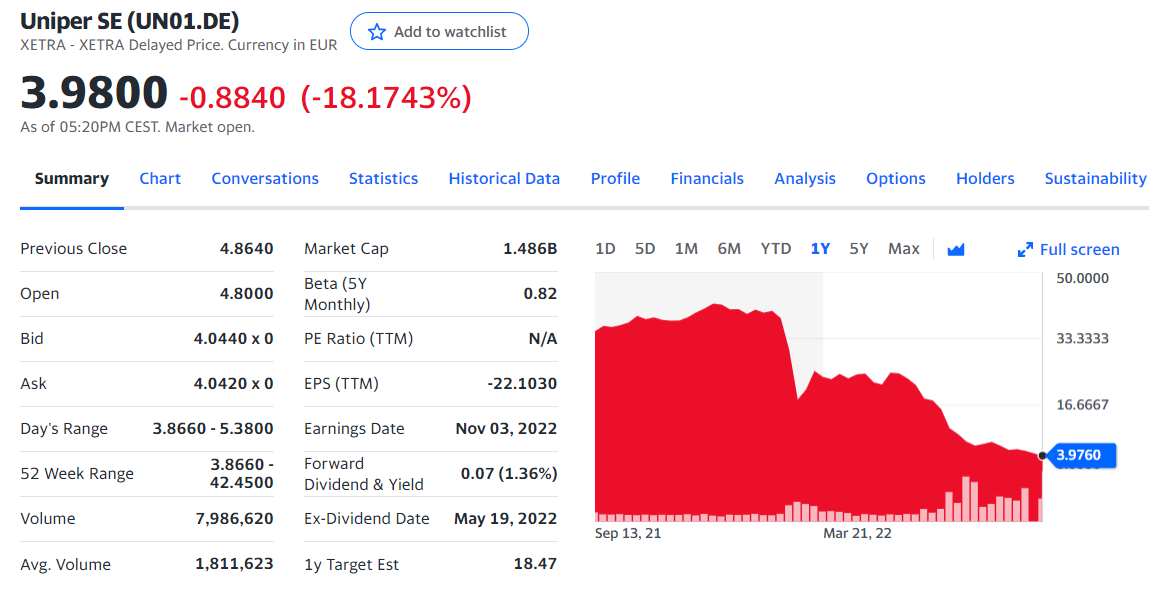**Detailed Stock Information for Uniper SE**

The image displays financial information on a white background with black and blue text, focusing on Uniper SE. The top left corner of the image features the company's name, "Uniper SE," followed by the annotation "Xetra Delayed Price. Currency in EUR (EUR)." Below that, the currently highlighted value is "3.9800," indicative of a current stock price.

Directly beneath the current price, the term "Summary" is underlined, suggesting it's an active selection, possibly from a menu or a tab. Various stock-related figures are listed, resembling a detailed financial report:

- **Previous Close**: 4.8640
- **Open**: 4.80
- **Bid**: 4.04
- **Day's Range**: (specific values not mentioned)
- **52-Week Range**: (specific values not mentioned)
- **Volume**: (specific values not mentioned)
- **Average Volume**: (specific values not mentioned)
- **Market Cap**: 1.486 billion (1.486B)
- **Beta (5Y Monthly)**: (value not mentioned)
- **PE Ratio**: (value not specified)
- **Earnings Date**: November 3rd, 2022

In the bottom right corner, there is a graph illustrating the performance of Uniper SE’s stock over time. The timeline on the graph spans from September 13th to March 22nd, and it depicts a downward trend in the stock price during this period.